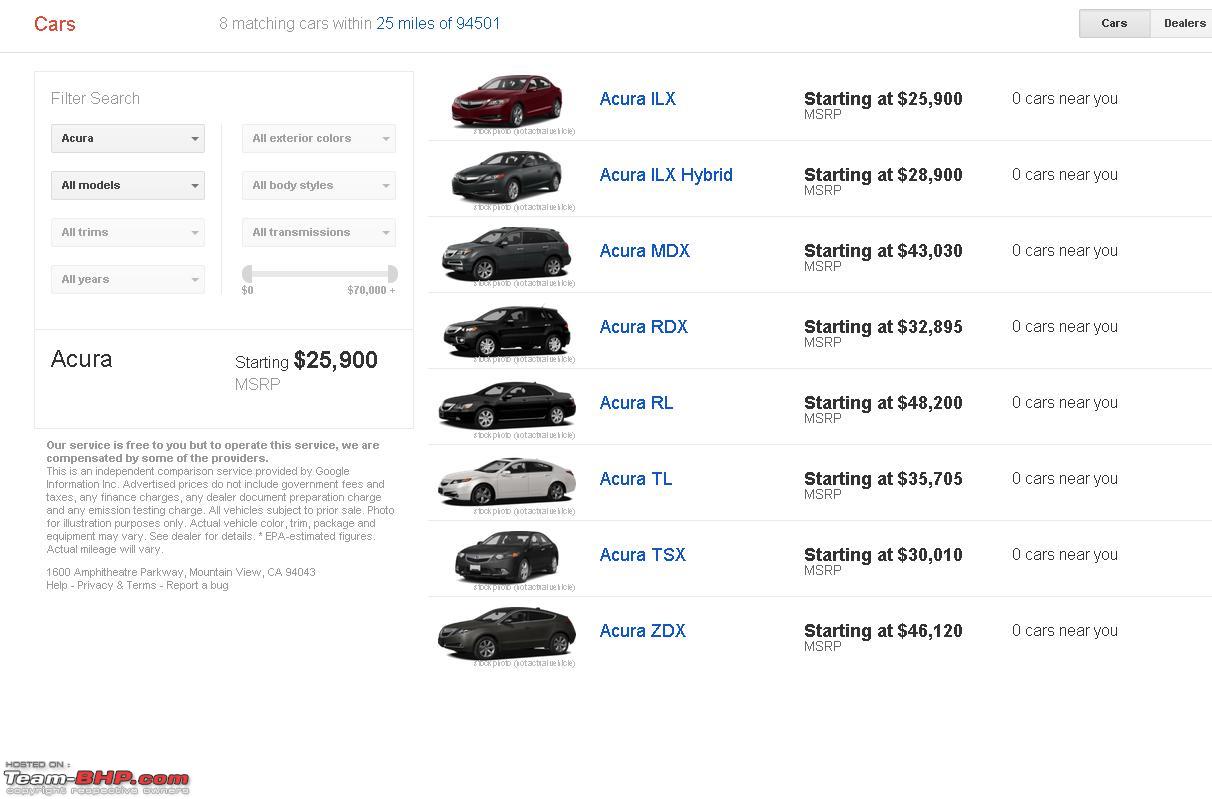The image depicts a screenshot of a web page dedicated to listing available cars. The page has a clean, white background without any borders. In the upper left-hand corner, the title "Cars" is prominently displayed in red text. Next to this, the page indicates that there are eight matching car listings available within 25 miles of the 94501 ZIP code. 

On the upper right-hand corner, there are two navigational buttons labeled "Cars" and "Dealers." Along the left side of the page, there is a comprehensive filter search box allowing users to refine their search based on brand, model, trim, body style, exterior colors, and transmission type. Below the filter options, the text "Acura starting $25,900 MSRP" is displayed, giving an introductory price point. 

Accompanying this section is a small area of additional text, and in the lower-left corner, the logo and text "hosted on teambhp.com" is evident, indicating the hosting website. 

The main body of the web page lists eight Acura models, each with corresponding images, names, starting prices, and availability. Despite the listings, it is noted that there are zero cars near the user for all models. The Acura models listed from top to bottom are:

1. Acura ILX
2. Acura ILX Hybrid
3. Acura MDX
4. Acura RDX
5. Acura RL
6. Acura TL
7. Acura TSX
8. Acura ZDX

The starting prices for these models range from $25,000 for the Acura ILX to $48,200 for the Acura RL.